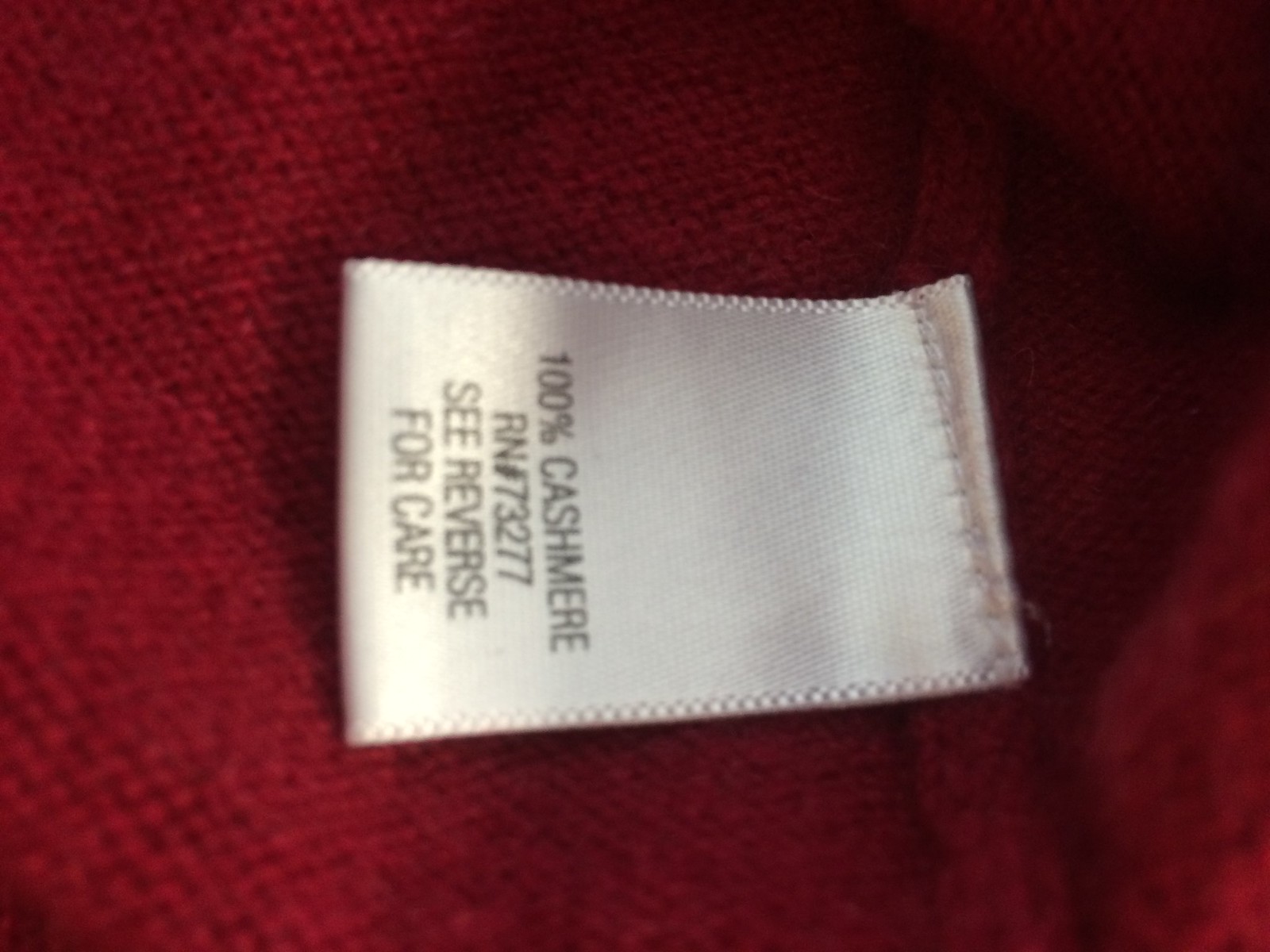This image showcases a detailed close-up of a tag on an article of clothing, which appears to be a reddish-maroon, possibly cashmere sweater. The luxurious fabric has a distinct sweater-like weave visible around the tag. The tag itself is positioned in the center of the image and is secured with red thread that matches the garment, displaying meticulous stitching along all sides. The white tag has black lettering with "100% cashmere," "RN 73277," and "See reverse for care" printed in what seems to be a capitalized Arial font. Notably, the tag lies on its side, requiring a tilt to the right to read the information clearly.